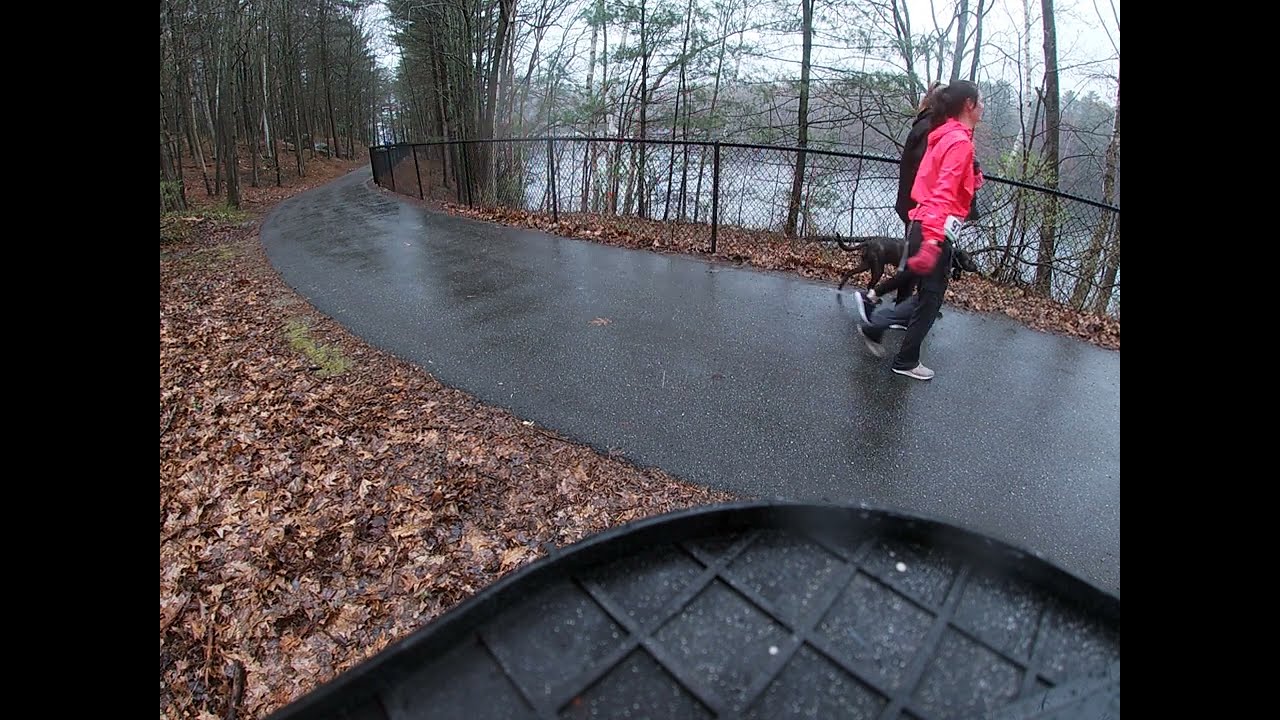In this detailed color exterior daylight photograph, a wet, black asphalt walkway winds through a fall landscape covered in brown, fallen leaves. The path, glistening from recent rain, curves gently into a forested area lined with tall, thin-trunked trees. In the foreground, a curious black grid-shaped object, possibly part of a textured step or a garbage can lid, appears on the ground.

Two women walk along the path. The closer woman sports a bright bubblegum pink jacket, matching gloves, black pants, and white shoes. Her brown hair is pulled back into a ponytail. Beside her, a woman with longer, lighter brown hair is dressed in a black jacket, black pants, and black sneakers with white soles. They’re accompanied by a large brown dog.

Flanking the path is a chain-link fence, behind which lies a serene lake, possibly frozen, adding an additional layer of tranquility to the composition. The entire scene, bordered by black bars on the left and right, frames the wet, autumnal beauty of the park setting.